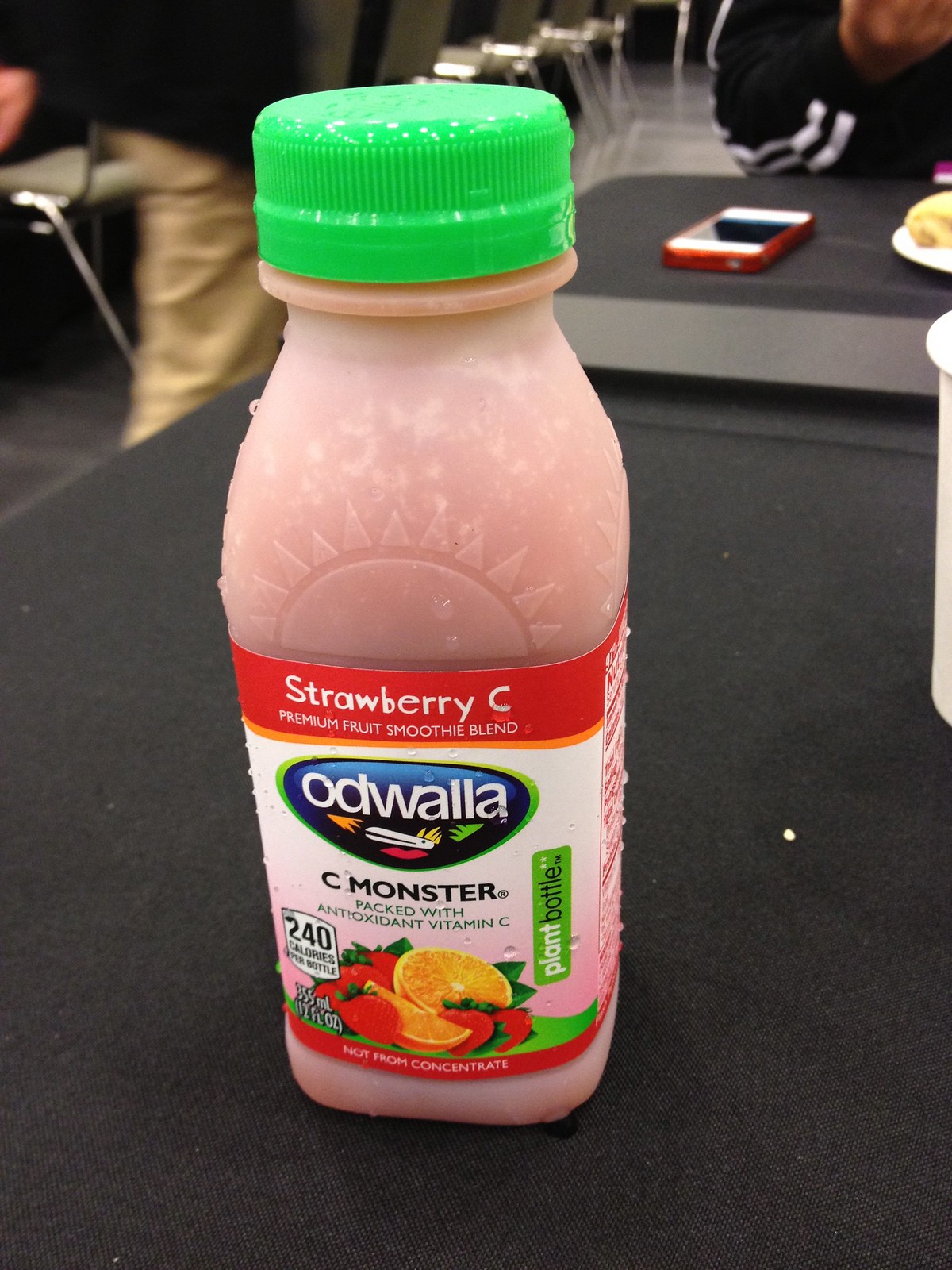This photograph features a bottle of Odwalla's Strawberry C Monster Premium Fruit Smoothie Blend prominently placed at the center of a table. The smoothie, rich in antioxidant vitamin C, comes in a semi-opaque, creamy-colored plastic bottle adorned with a vibrant green cap. The label on the front showcases an enticing illustration of fresh strawberries alongside a whole and a sliced orange, conveying the fruity flavor of the smoothie. The bottle also highlights key information such as "240 calories" and "plant bottle," emphasizing its nutritional content and eco-friendly packaging. In the background, there are people seated around the table and an iPhone with a red case is noticeable among other trivial items, adding a sense of everyday context to the setting.